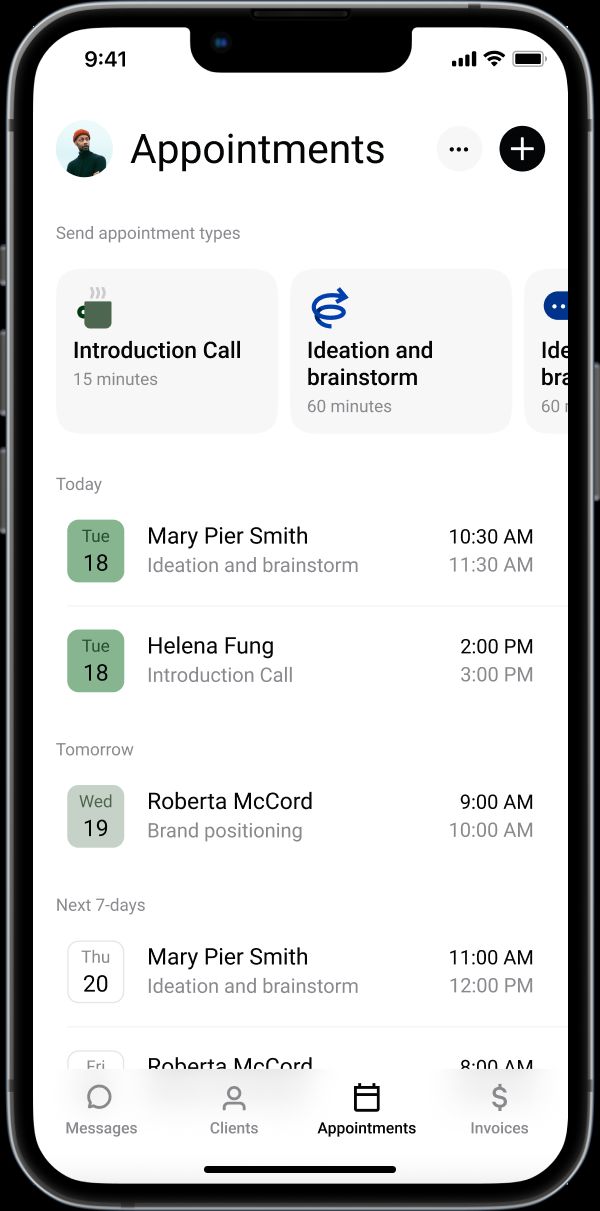The image displays a smartphone screen with a black outline. At the very top, the status bar shows the time as 9:41, Wi-Fi signal strength with four bars, the Wi-Fi icon, and a full battery indicator. Below the status bar is a section featuring a person's profile picture and the word "Appointments." To the right of this, there are three vertical dots indicating more options and a plus sign enclosed in a black circle for adding new appointments.

In lighter text, the screen reads "Send appointment types," and below it, there is a coffee cup icon next to the label "Introduction Call," which has a duration of 15 minutes. Adjacent to this is a shaded box labeled "Ideation and Brainstorm," indicating 60 minutes in duration.

Further down, a calendar layout starts with "Tuesday the 18th" showing two appointments. Then it lists "Wednesday the 19th, tomorrow," and "Thursday the 20th" for the next seven days, although only part of the next line is visible. Specific appointments are detailed below these dates:
- Mary Pierce-Smith: Ideation and Brainstorm at 10:30 AM on the 18th.
- Helena Fung: Introduction Call at 2:00 PM on the 18th.
- Roberta McCord: Brand Positioning at 9:00 AM on the 19th.
- Mary Pierce-Smith: Ideation and Brainstorm at 11:00 AM on the 20th. 

This structured schedule is neatly organized, providing a clear overview of the upcoming meetings and their details.